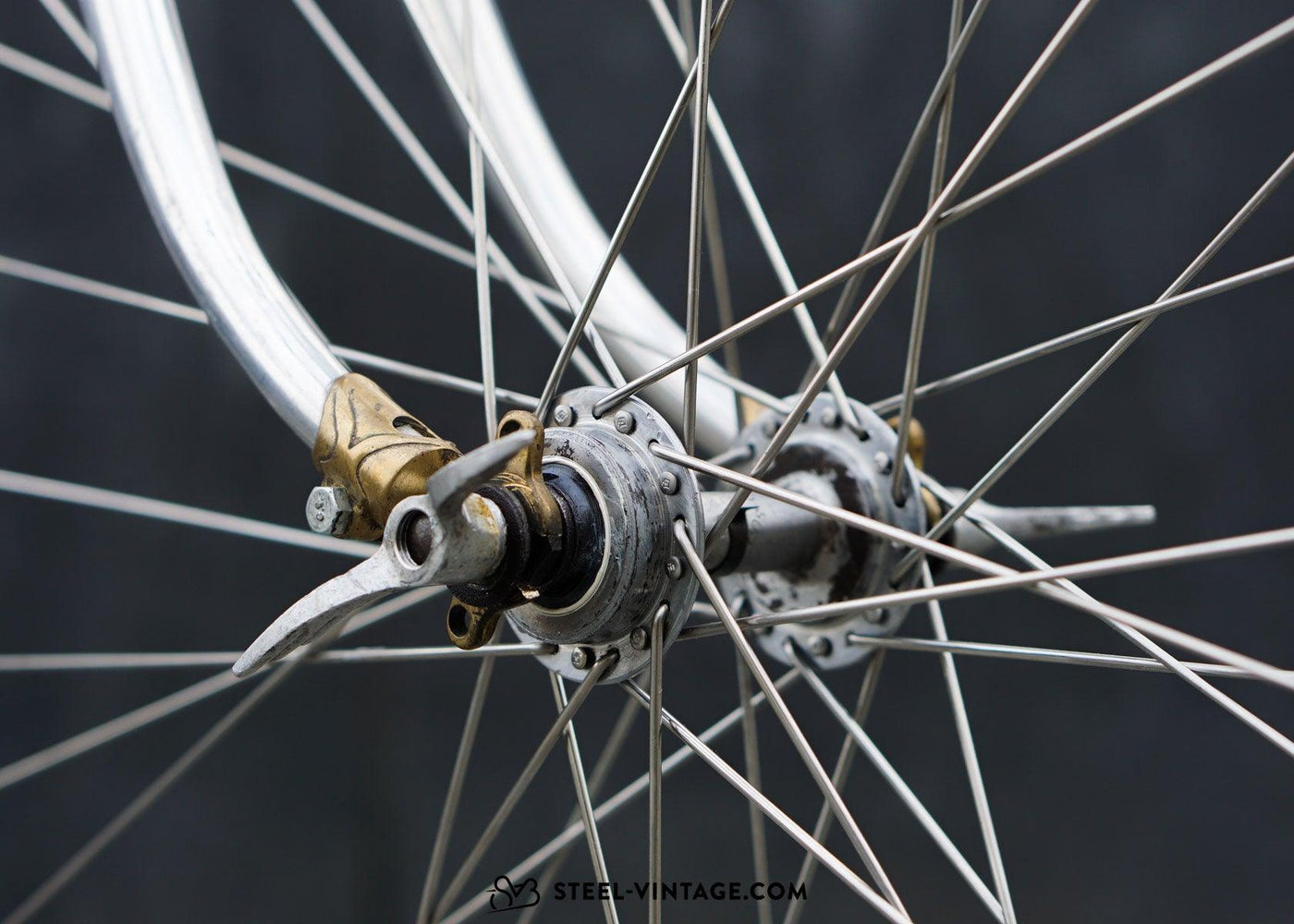A close-up photograph captures the intricate details of a bicycle wheel's hub and spokes. At the center, a cylindrical hub is flanked by two circular plates, each secured with several black bands and a prominent bolt. Radiating from this hub, a network of silver-toned spokes extends outward to connect with the wheel's rim, set against a dark gray background that enhances their clarity. A thicker, silver-toned section of pipe with a brass covering adds a contrasting element to the composition. Centered at the bottom of the image, the text "SteelVintage.com" is prominently displayed.